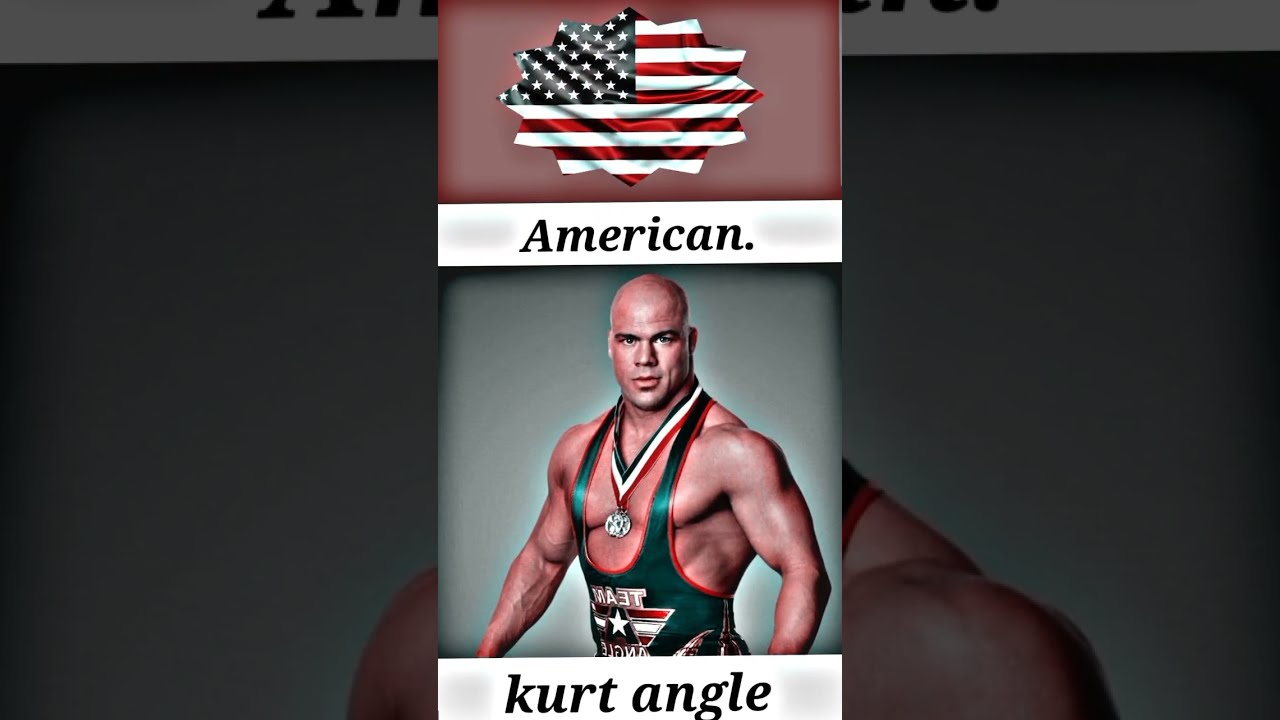The image features a muscular, bald man identified as Kurt Angle, who is dressed in a wrestling uniform. His outfit is a distinctive blue tank top with a red border that awkwardly exposes his chest and is emblazoned with the words "Team Angle" in red and white stripes, accompanied by a white star on a blue background. Interestingly, the text on the outfit appears backwards. He is also wearing a silver medal with a red, white, and blue neckband. The top section of the image includes a jagged cutout revealing part of the American flag with multicolored stripes peeking through a brownish background. Above the picture of Kurt Angle, a white banner with black text reads "American," while a similar banner below his image spells out his name in lowercase letters, "kurt angle." Both his facial expression and the text orientation add a slightly peculiar touch to the composition.